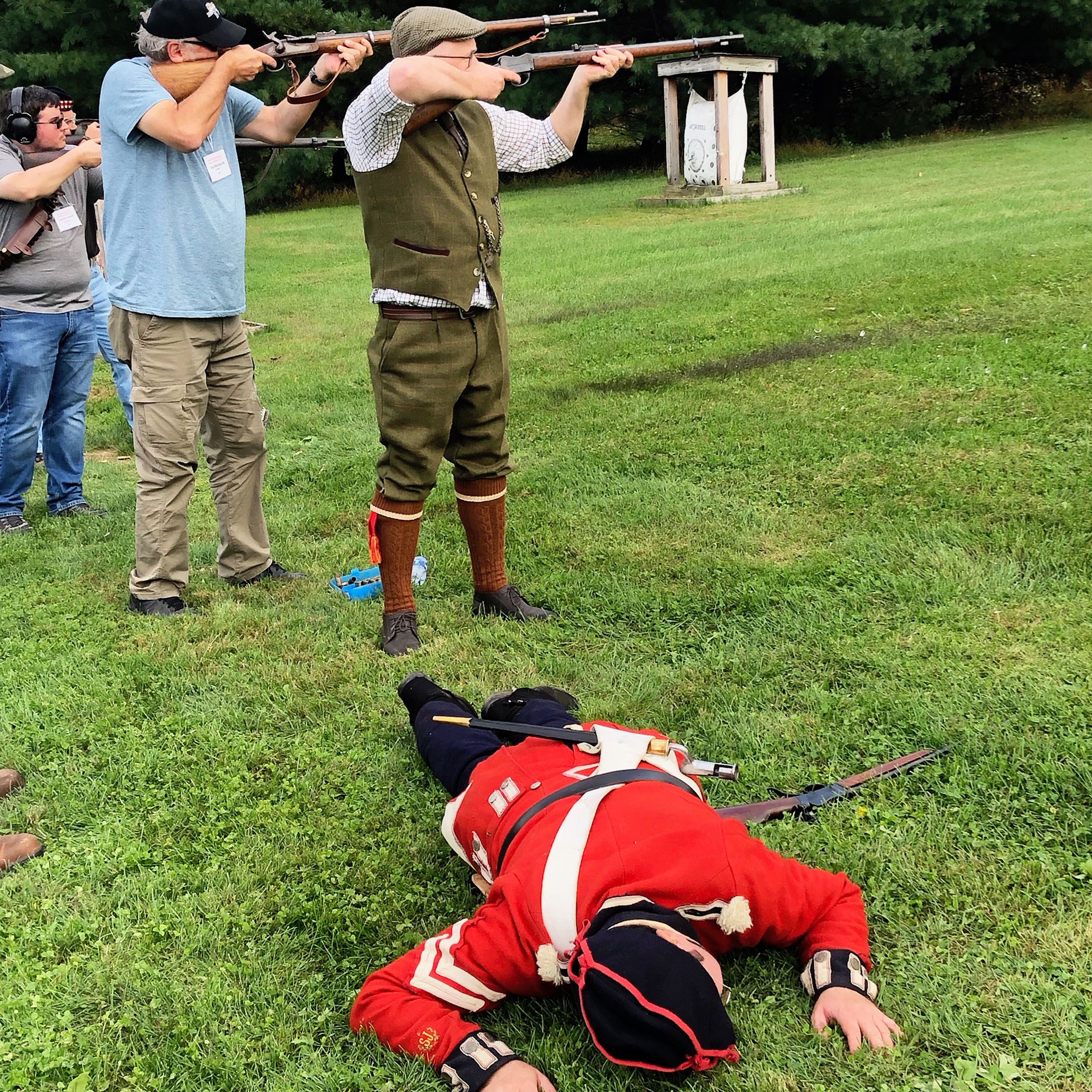In the photograph, there is a well-maintained lawn where three Caucasian men are standing, each holding a long rifle pointed forward. The first man, dressed in a dark green beret, green vest, green shorts, and brown knee-high socks, has a rustic, outdoor appearance. The second man wears a blue t-shirt, khaki pants, and a black baseball hat, while the third man sports a light gray t-shirt, jeans, over-the-ear headphones, and sunglasses. In front of these men lies a person in a striking red and black uniform, reminiscent of a military or Scottish attire. This prone figure, face down, is adorned with a red jacket featuring black cuffs with white markings, black pants, and a black and red cap, along with a ribbon across his back and stripes on his right shoulder, indicating a rank. Despite the odd positioning, the three standing men seem to pay no attention to the individual on the ground, adding an element of intrigue to the scene.